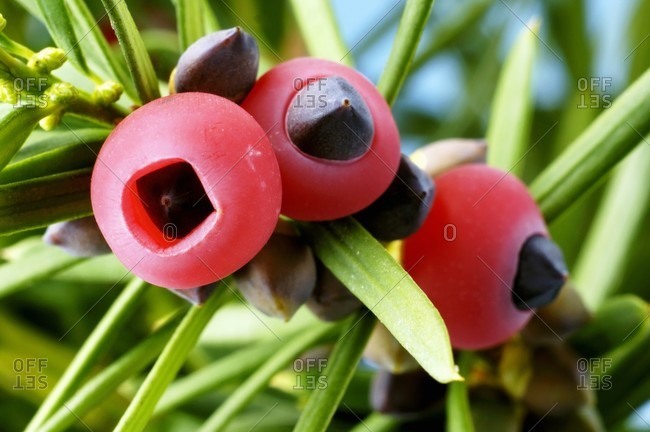This close-up stock photograph features a striking red fruit growing on a green plant with tiny, pointy leaves. The fruit, small and about half an inch in diameter, is red with a central, dark purple-black seed which can be seen through the semi-translucent, fleshy outer layer. Some of the fruits in the image show just the black seed, either because the red outer part has fallen off or hasn't yet formed. The plant and its vividly colored fruit are the focal points, set against a blurred background that hints at additional greenery and a faint blue sky. The image has several watermarks, repeating the word "offset" along with thin hash lines across the photo, indicating its stock photograph nature. The vividly juxtaposed colors of red, green, and black make the fruit stand out sharply, capturing attention with its exotic appearance.